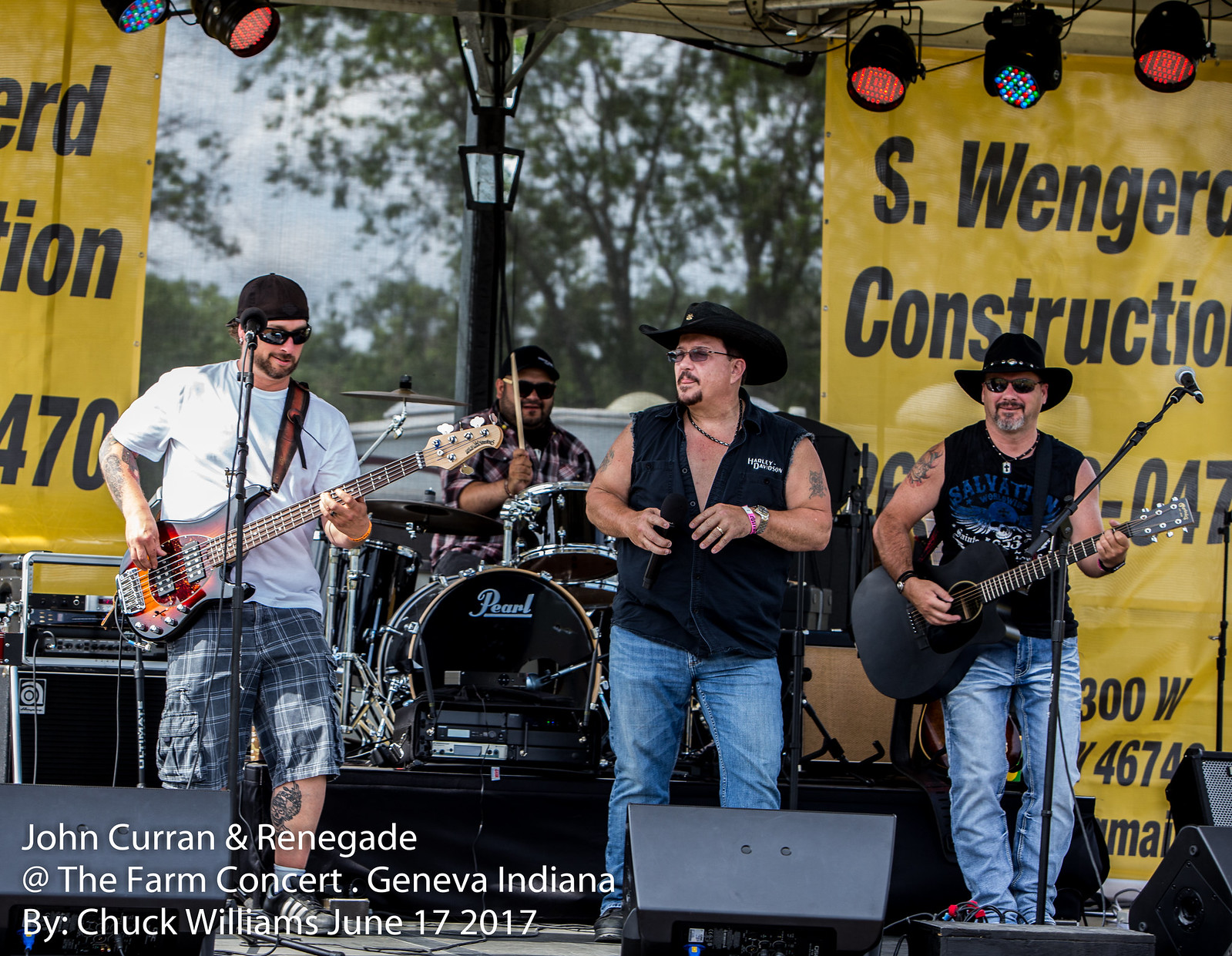The image captures an outdoor concert featuring a country-western rock band on stage. The stage is adorned with two large yellow banners reading "S. Wengerd Construction." At the far left, a guitarist is seen wearing a white t-shirt, blue shorts, black baseball hat, black sunglasses, and playing a guitar. Next to him is the drummer, positioned behind a black drum set, dressed in a black hat, sunglasses, and a flannel shirt. Moving to the right, the lead singer stands at the center holding a microphone in his right hand, sporting a black cowboy hat, black sleeveless vest, blue jeans, and sunglasses, with a watch visible on his left wrist. The acoustic guitarist on the far right is also dressed in blue jeans, a black cowboy hat, sunglasses, a black short-sleeved shirt, and is engaged in playing a black guitar. In front of the stage, there are several speakers, while the background reveals scenic elements like trees and the sky. A watermark at the bottom left reads "John Curran and Renegade at the Farm Concert, Geneva, Indiana by Chuck Williams, June 17, 2017."